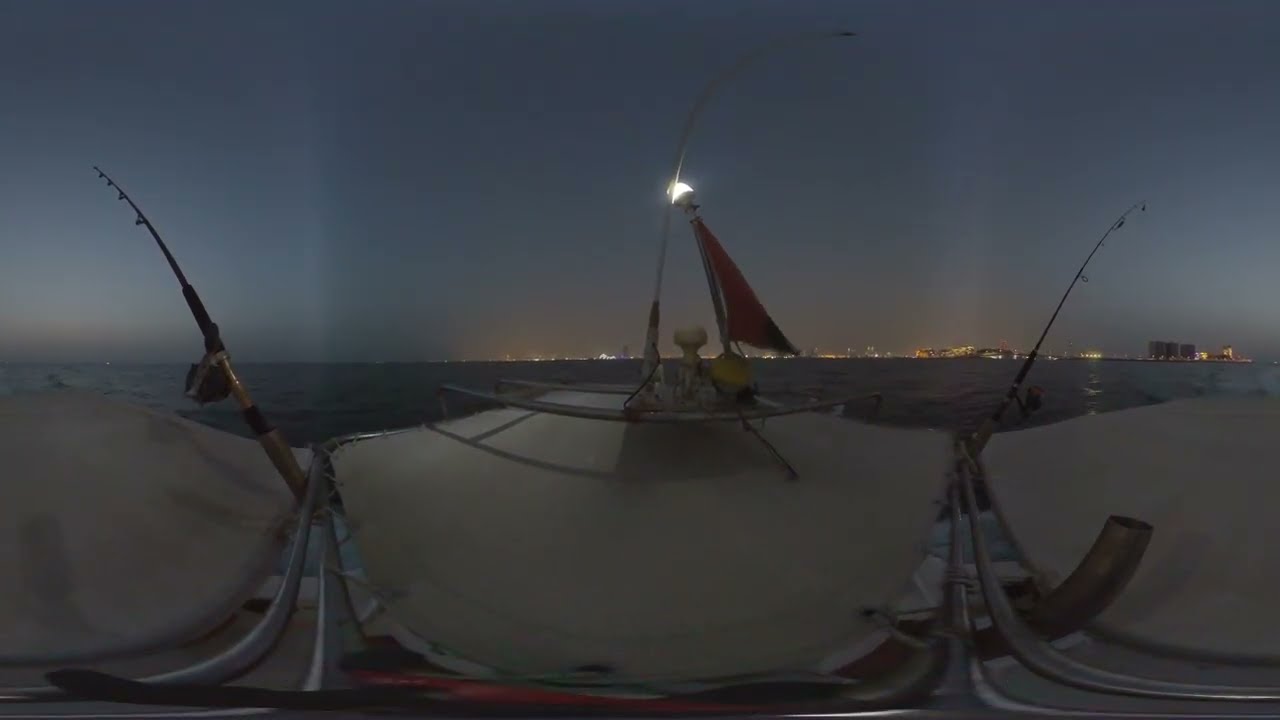This photograph captures the view from the front of a sailboat as it navigates through the ocean at dusk, with the sky transitioning into a deep blue haze. In the foreground, white panels, resembling the shape of shields, are mounted on metal posts, possibly serving as part of the boat's structure. Fishing rods are strategically placed on both sides and one in the center, their lines cast into the water. A red sail is faintly visible under the dim night sky, and a small white light can be seen at the top of the sail, providing illumination. The distant horizon reveals the glow of city lights, possibly marking the location of a harbor, guiding the boat back home as night falls.